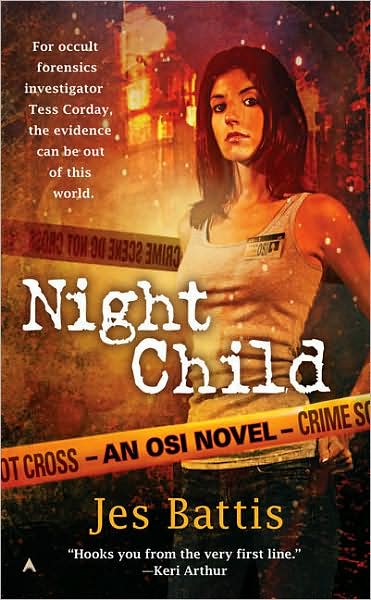The cover image of the book "Night Child" by Jess Battis prominently features a young woman with shoulder-length brown hair and an intense gaze, dressed in a sleeveless white tank top and jeans. The scene depicts her standing against a city backdrop, partially obscured by yellow crime scene tape marked with "Do Not Cross". In the top left corner, the white text reads, "For Occult Forensics Investigator Tess Corday, the evidence can be out of this world." Below the title "Night Child" in bold white font, the author's name, Jess Battis, appears in yellow text. Further down, a quote from Kerry Arthur in white text states, "Hooks you from the very first line." In the background, a building seems to be on fire, adding to the dramatic and suspenseful atmosphere portrayed on the cover.